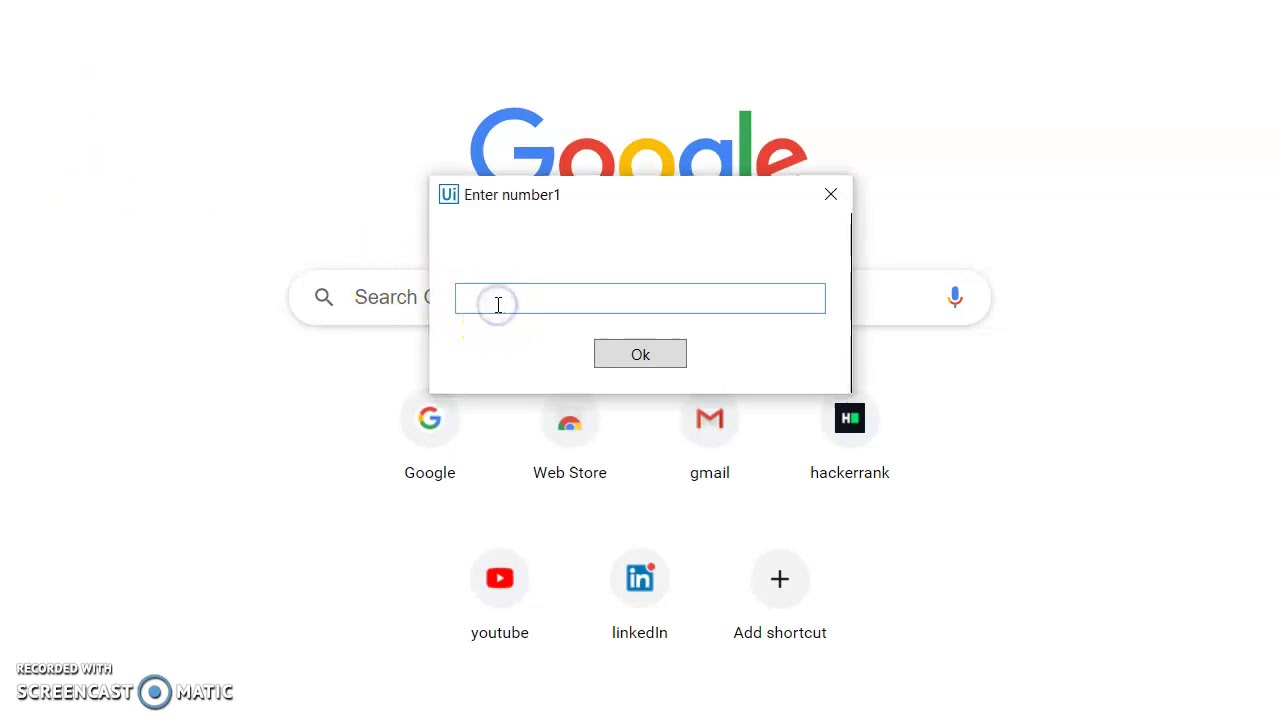The screenshot captures a Google Search page with a pop-up dialog box in the foreground. The dialogue box, which occupies the center of the screen, prompts the user to "Enter number one." The UI design of the box includes a faint circular highlight around the input field, indicating where text can be typed. Positioned at the bottom of the box is an "OK" button, rendered in gray.

In the background, the Google Search page features the iconic Google logo in its rainbow colors: blue for the 'G,' red and yellow for the 'O's, green for the 'L,' and blue again for the 'E.' Below the search bar, a selection of recently used applications and shortcuts are visible, including "Google Web Store," "Gmail," "HackerRank," "YouTube," "LinkedIn," and an option to "Add shortcut."

Additionally, in the bottom-left corner of the screen, the icon for "Screencast-O-Matic" is present. This tool is designed for screen recording, allowing users to create video guides by narrating their on-screen activities. The overall image effectively showcases a typical Google Search interface, interrupted by the aforementioned dialog box prompting user interaction.